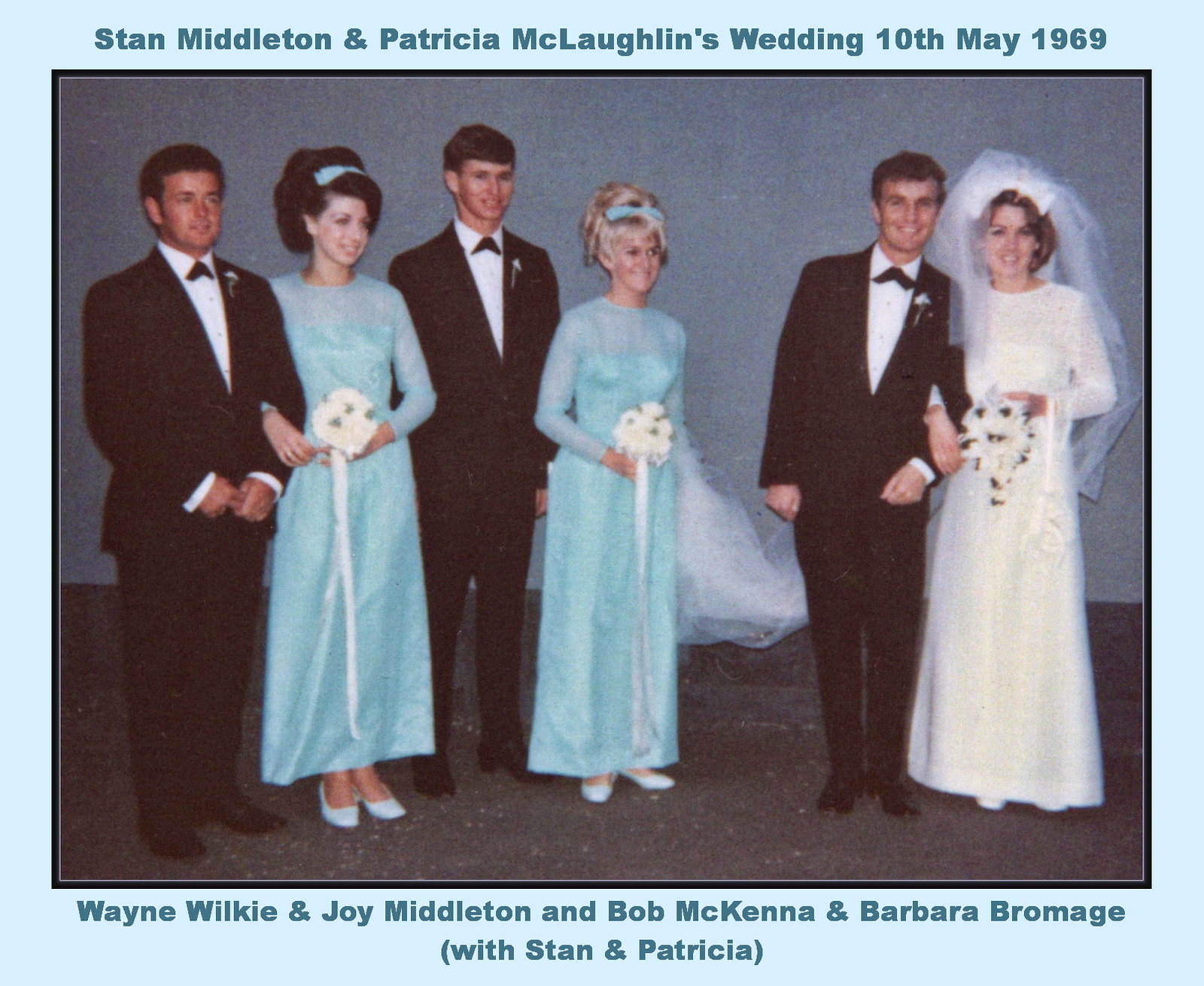The image, surrounded by a light blue border with dark blue text, captures the wedding of Stan Middleton and Patricia McLaughlin on 10th May 1969. The top inscription reads "Stan Middleton and Patricia McLaughlin's Wedding, 10th May 1969," while the bottom lists the names Wayne Wilkie and Joy Middleton, and Bob McKenna and Barbara Bromage alongside "Stan and Patricia."

The photograph features three couples, with the bride and groom positioned on the right. The groom, standing just left of the bride, is in a traditional black tuxedo paired with a white shirt and black bow tie. He slightly leans towards his bride, who is adorned in a classic white wedding dress and a flowing lace veil that extends behind her. She holds a white bouquet of flowers, clasped in front of her midriff.

To the left of the bride and groom stand the other two couples: first a man and a woman, then another man and woman. Both men match the groom in black tuxedos. The bridesmaids wear elegant light blue dresses that reach down to their ankles, paired with matching light blue shoes and holding smaller white bouquets accented with white ribbons. The visual harmony and formal attire emphasize the celebratory and intimate nature of the occasion.